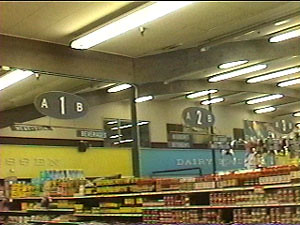The photograph captures an interior view of a grocery store. The ceiling and walls are beige, providing a neutral backdrop to the scene. Strobe lights are visible on the ceiling, illuminating the area. Overhead, large signs demarcate the different aisles: the first sign reads 'A' on the left, '1' in the middle, and 'B' on the right; the second sign displays '2' with 'A' to its left and 'B' to its right; similarly, the third sign shows '3' with 'A' on the left and 'B' on the right. The aisles contain various products: aisle '1A' seems stocked with condiments such as hot sauce, pickles, and assorted seasonings like salt and pepper. There's also a selection of sauces that might include spaghetti sauce. The floor isn't visible in this image, focusing the viewer's attention on the structured layout and stocked shelves of the grocery store.